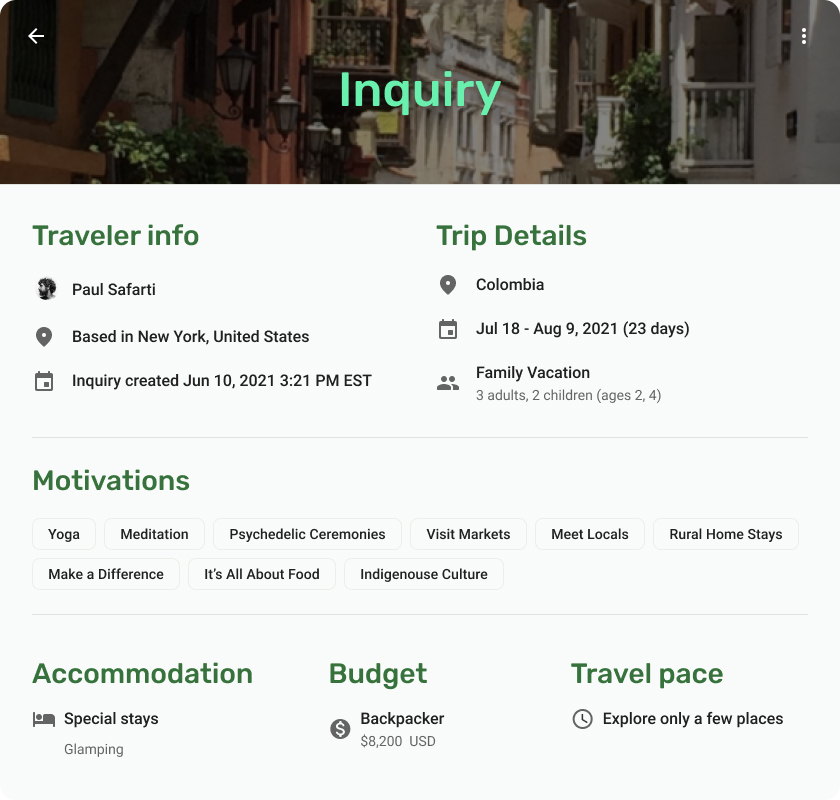The image features an inquiry for a vacation trip to Colombia, initiated by Paul Sephardi from New York, United States. The top banner showcases an image of a building, possibly resembling a hotel or apartments, with the word "Inquiry" prominently displayed in lime green text. Below this, against a white background, it reads:

**Traveler Info:**
- **Name:** Paul Sephardi
- **Location:** Based in New York, United States

**Inquiry Details:**
- **Created On:** January 10th, 2021 at 3:21 PM Eastern Standard Time
- **Trip Destination:** Colombia
- **Travel Dates:** July 18th through August 9th, 2021
- **Duration:** 23 days
- **Participants:** Family Vacation for three adults and two children (ages two and four)

**Travel Motivations:**
- Yoga
- Meditation
- Psychedelic Ceremonies
- Visiting Local Markets
- Meeting Locals
- Rural Homestays
- Emphasis on Food and Indigenous Culture

**Accommodation Preferences:**
- Budget: Backpacker style with a total budget of $8,200
- Travel Pace: Prefers to explore a few selected places

This detailed description encapsulates the individual’s comprehensive trip itinerary and preferences for their vacation in Colombia.